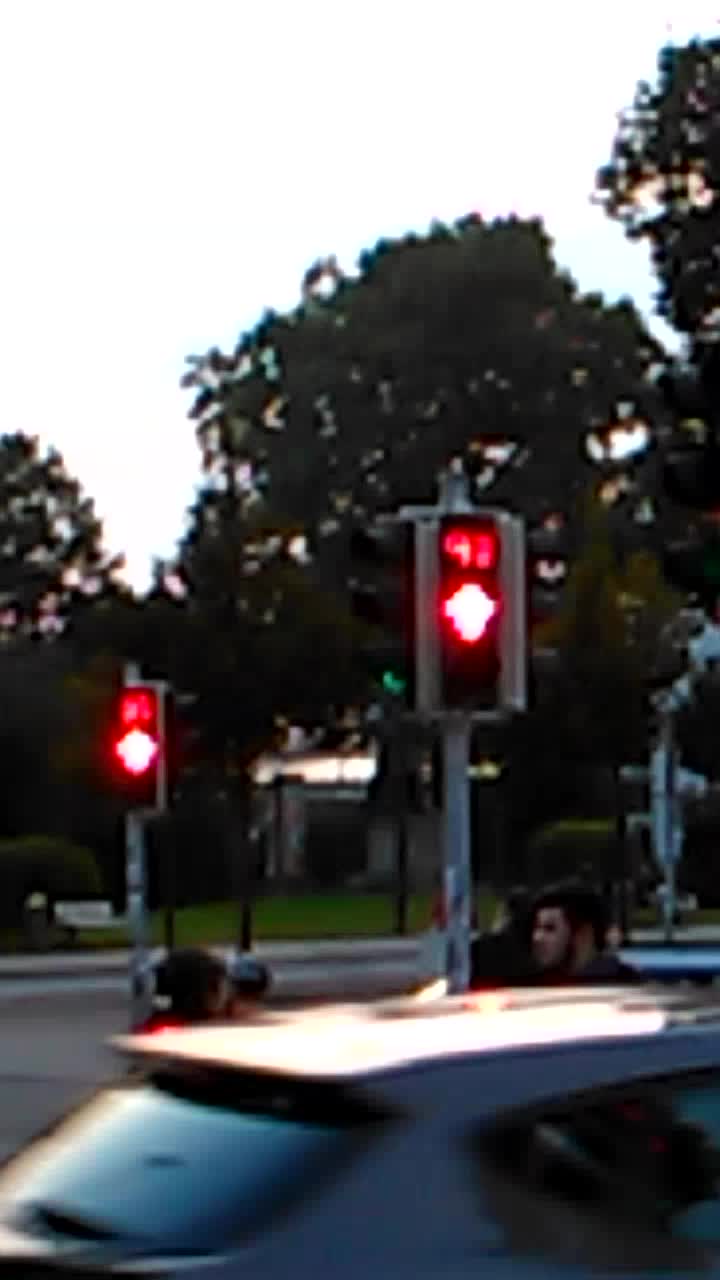This blurry photograph depicts a street corner scene, characterized by two indistinct speed limit signs and red stoplights. In the foreground, a mid-sized sedan with dark tinted windows is prominently visible, with the top of the car’s roof gleaming under low light conditions. The car is positioned from left to right, revealing the back window on the left and the side window on the right. Just above the car, you can see the heads and upper shoulders of two or three individuals. One figure, with dark hair and a red shirt, is visible above the back windshield, while another man with short hair and a beard is on the right side above the hood, looking to the right. A silver pole with a rectangular sign featuring indiscernible red numbers and a blurred yellow section stands in front of him. Additional trees line the background, stretching halfway up the image, with a grayish building faintly visible through the foliage. The sky above the trees is a pale blue, while the overall light suggests early morning or late evening. Off to the far left edge of the image, another similar pole with traffic signs is almost off-frame. A white park bench can also be seen across the street.